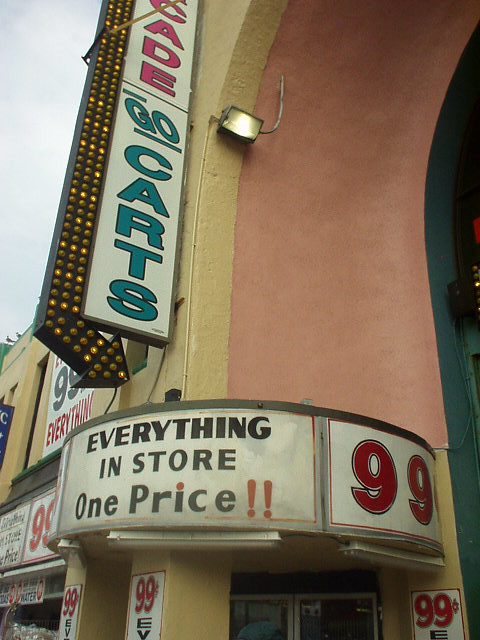This image depicts the exterior of a large, Art Deco-style building characterized by its cream and peach stone facade, accentuated with green highlights on the left side. At the top center of the structure is a partially visible, neon-lit white sign that begins with the letters "C-A-D-E," suggesting it initially spells "arcade." Accompanied by a black line, the sign also features the green-lit words "go-karts" with horizontal lines above and below the "G" and "O." 

Beneath this main sign is an illuminated arrow composed of multiple lights, pointing downward toward the entrance, marked by a bold red "99" and words declaring "everything in store, one price," followed by two red exclamation marks. Prominently featured throughout the facade are red "99 cents" symbols, emphasizing the recurring theme of uniform pricing. The building's arched top houses two large glass doors framed in silver metal, hinting at the main entrance. The overall visual presentation is vibrant with elements in red, green, and various shades of cream and peach, creating a striking and colorful storefront.